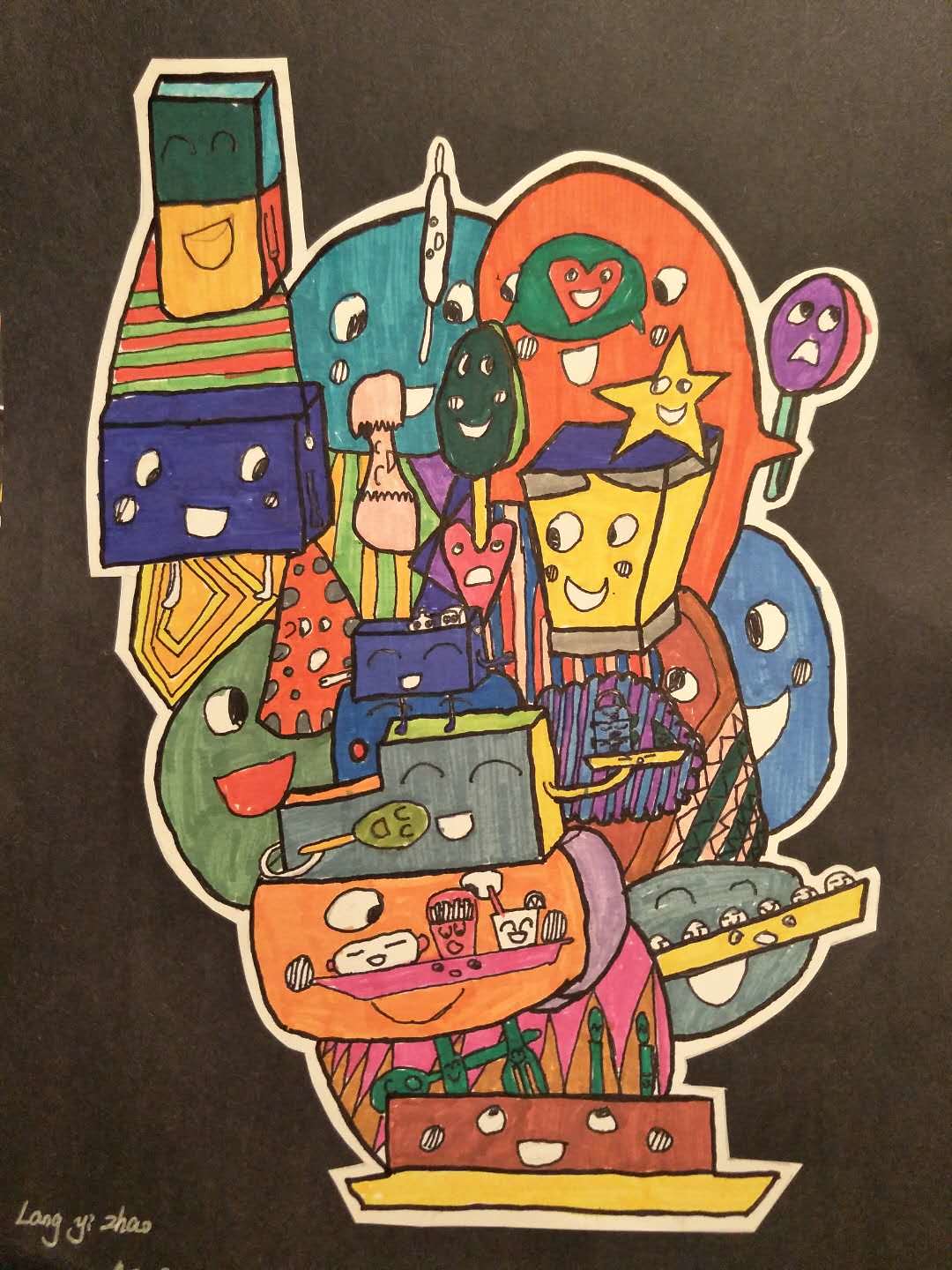This artwork, vividly colored with markers, features an array of geometric shapes, each adorned with charming, cartoonish faces. It appears to be meticulously cut out and mounted on a dark, rectangular background, possibly black or dark brown-green. The image includes numerous shapes such as boxes, triangles, stars, and circles, all with white eyes and open mouths. Some faces are decorated with blushing cheeks, and most are smiling. The shapes are rendered in a variety of vibrant primary colors, stacked and layered upon one another, creating a dynamic and cheerful composition. Notably, figures resembling characters like SpongeBob SquarePants, a hamburger, and a lollipop are part of this playful ensemble. The artist, Yi Zhao, has signed the piece in the lower left corner, adding a personal touch to this expressive, joyful creation.